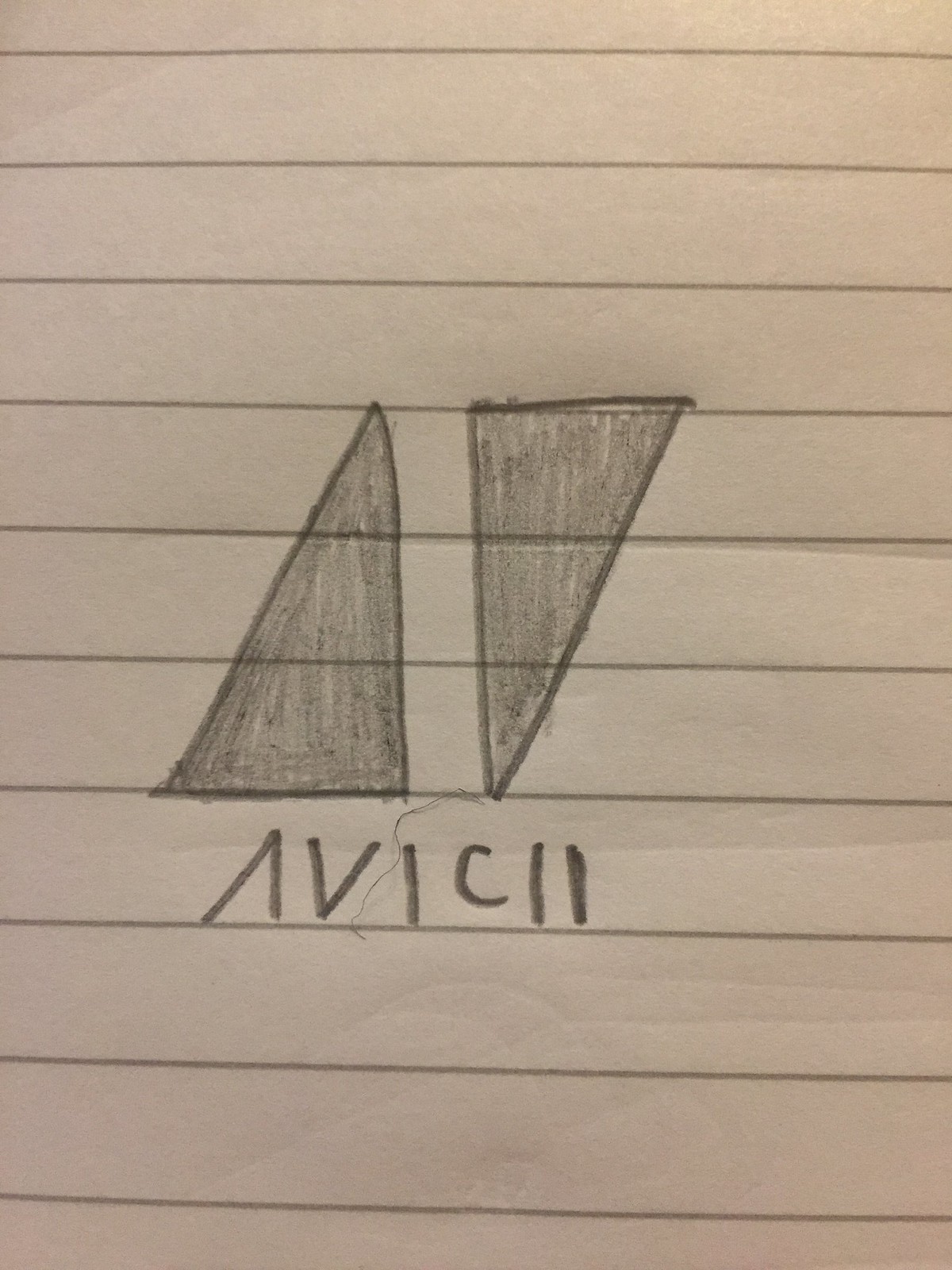This image shows a piece of lined paper, made from a thin material with an off-white, slightly grey hue. Dark grey horizontal lines traverse the page. While the paper is mostly crisp and flat, there is a noticeable crease in the top left corner and another horizontal crease about two-thirds of the way down. Additionally, there are subtle dents on the surface, suggesting someone drew on a sheet placed above this one.

In the center of the page, a pencil drawing captures attention. Two isosceles triangles are prominently featured. The first triangle points upwards, with its single vertex facing north. It has a thick pencil outline and is filled in with pencil, albeit in a slightly messy manner. Beside it, the second triangle is inverted, with its point facing downwards, and it mirrors the style of the first triangle.

Beneath these triangles, the word "Avicii" is written in pencil, mimicking the artist’s signature style. The overall composition pays homage to Avicii, captured on this intricately detailed piece of paper.